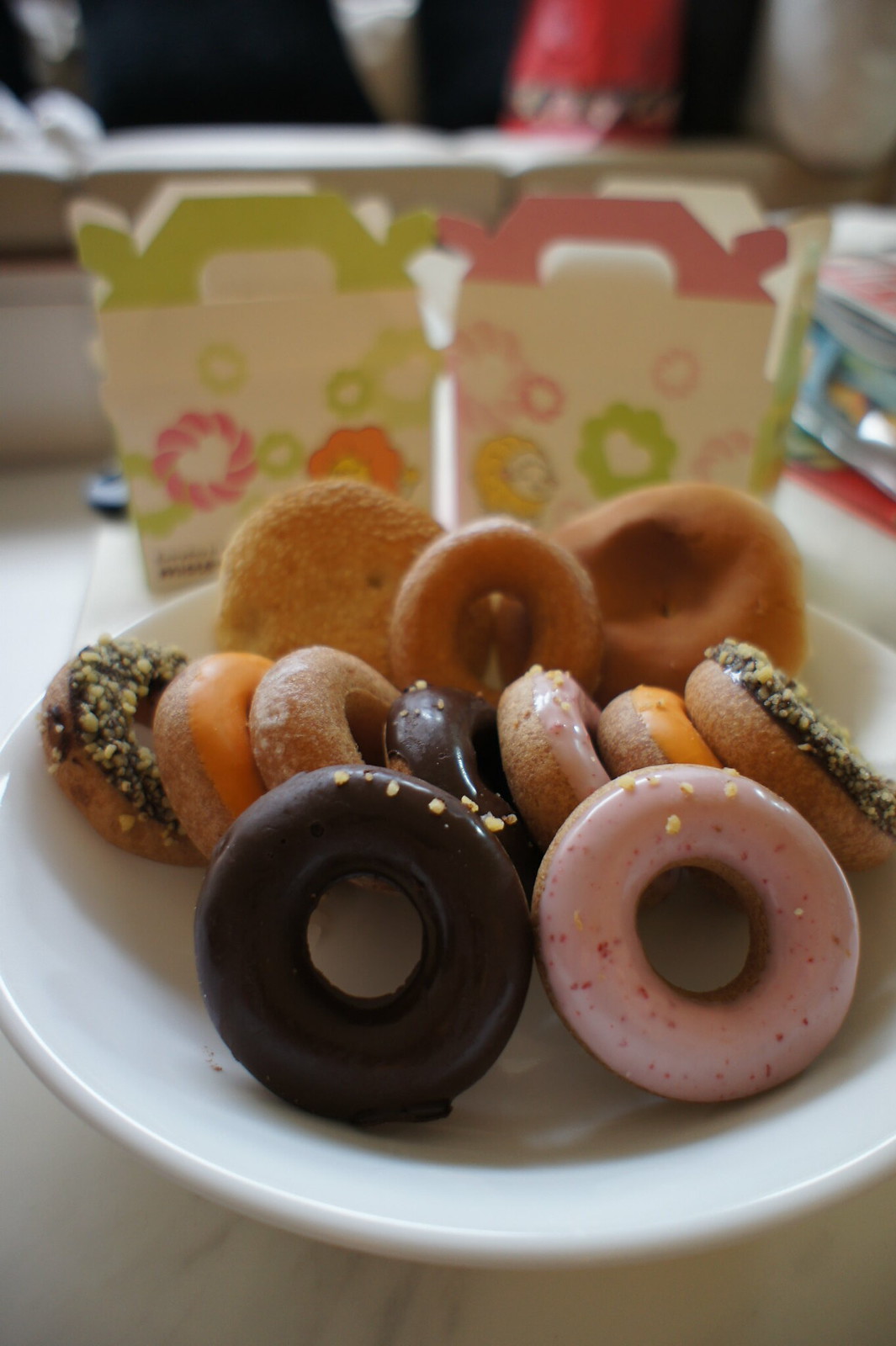In this delightful image, an array of twelve beautifully decorated donuts is presented on a plain white bowl-like plate. At the front center, a donut with pink strawberry frosting sits next to a chocolate-glazed donut. Behind them, a row of seven donuts recline partially atop one another, featuring a colorful mix of icing: chocolate, orange, pink, plain, and adorned with various toppings, including nuts and perhaps Butterfinger candy pieces. Toward the back of the plate, two additional donuts with holes flank another whole donut. 

This tempting arrangement is set against an off-white surface, and two ornate, fold-up to-go boxes stand prominently in the background. The left box is light green with white and green floral designs, complete with green handles, while the right box is pink with similar floral patterns and matching pink handles. The softly blurred background hints at a cozy indoor setting, possibly within a home or a café.